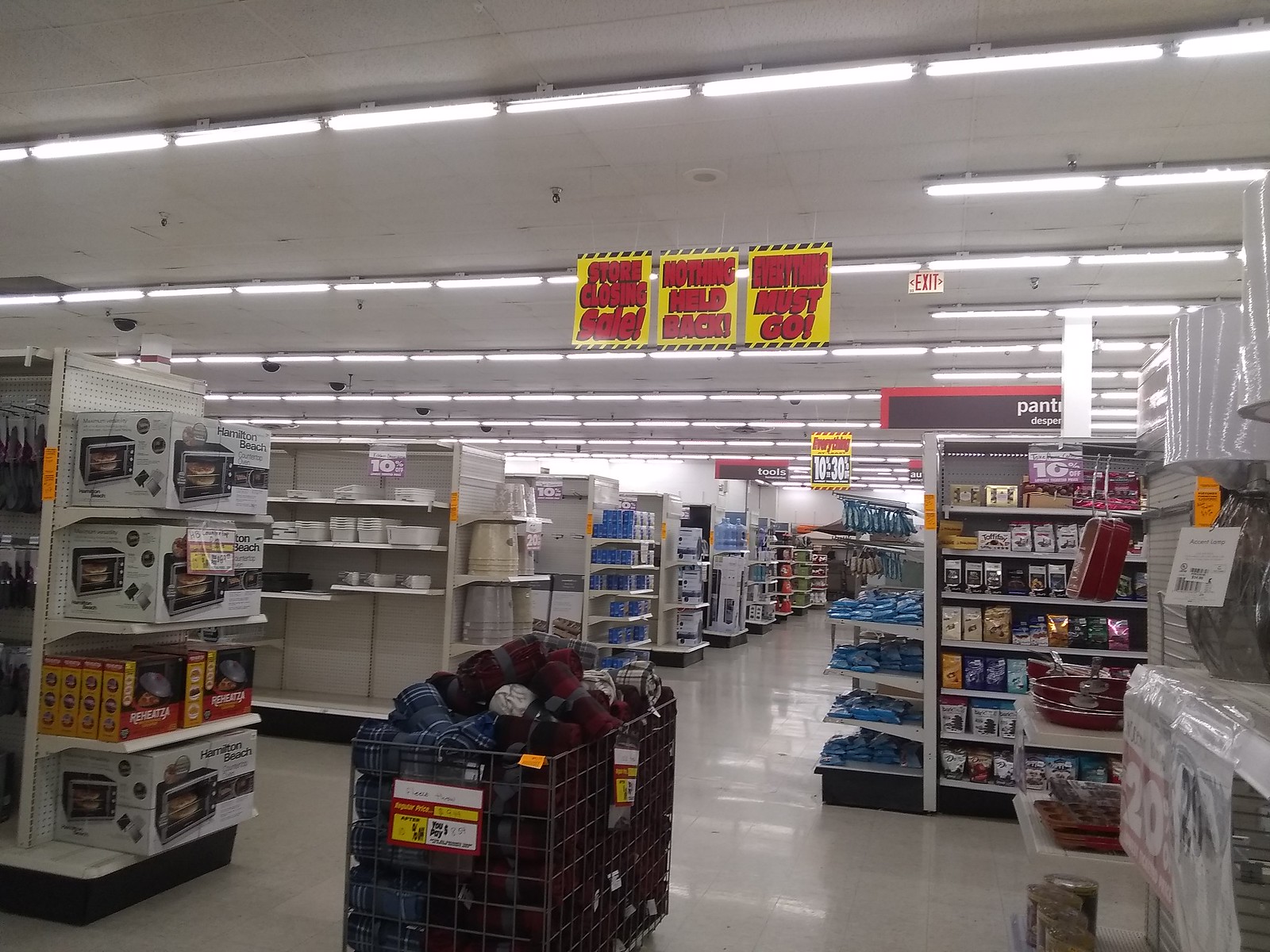This color photograph captures the interior of a department store taken in landscape orientation. The store is illuminated with bright lighting, accentuating details throughout the image. Dominating the scene are three prominent yellow signs with bold red lettering, each displaying urgent messages: "Store Closing Sale," "Nothing Held Back," and "Everything Must Go." Each sign is bordered by black dashes at the top and bottom, heightening their visibility and the sense of urgency.

The store appears partially picked over, with roughly 80% of the merchandise still on display. Some shelves, however, are noticeably emptier than others. The absence of shoppers gives the store a deserted feel, allowing the focus to be on the products, which include several toasters and a bin filled with blankets situated in the middle of the aisle. Additional sales signs are visible throughout, indicating discounts ranging from 10% to 30% off. The photograph provides a comprehensive view down an aisle, revealing a mixture of stocked and semi-empty shelves, reinforcing the impression of an ongoing store closure.